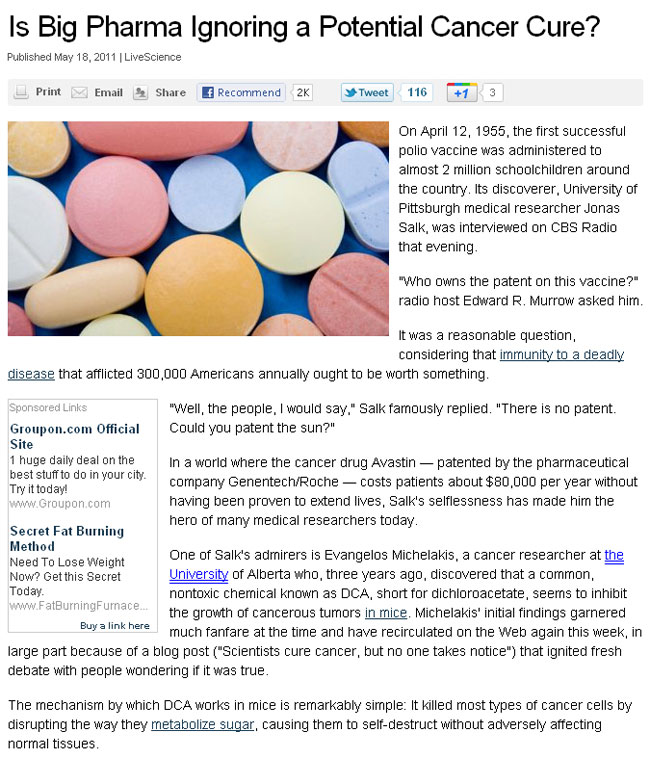This is a detailed caption describing a photo taken of a webpage from a newspaper website.

---

The webpage features a predominantly white background with large, black, capitalized lettering near the top left corner, extending almost completely across to the right. The headline reads, "Is Big Pharma Ignoring a Potential Cancer Cure?" Below this headline, in smaller black text, is the publication date, "Published May 18, 2011." A vertical dividing line separates this text from another section labeled "Life Science."

Below this, there's a gray border section. On the left side of this section, there are several icons: a print icon with the word "Print," an email icon labeled "Email," and a share icon marked "Share." To the right of these icons is the Facebook icon, next to which "Recommended" is written in blue, followed by "2K" in black lettering within a white square. Further to the right are the Twitter icon featuring a blue bird and the word "Tweet," with the number "116" beside it, and the Google Plus icon showing "+1."

The main content of the article is divided into a left and right segment. On the left is a prominent image displaying a variety of pills in different shapes, sizes, and colors, including purple, pink, yellow, blue, and orange. There appears to be approximately twelve pills featured in the photograph.

To the right of the image, the article begins with a paragraph that's about seven lines long, followed by a couple of lines of text, and then another three-line paragraph. Further down, a small rectangle labeled "Sponsored Links" appears, listing two links. The right column of the webpage continues with three more paragraphs of text, concluding the article's visible content.